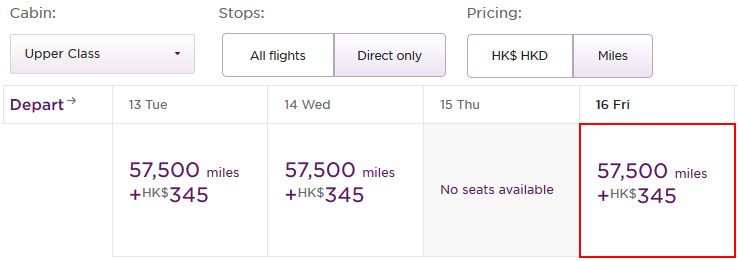The image depicts a flight booking website with a predominantly white background. Most of the text is in gray, with some light purple accents for key elements. The top section of the interface features three main categories:

1. **Cabin:** Located in the top left, this section has a drop-down menu, with the "Upper Class" cabin option selected by the user.
2. **Stops:** Positioned in the top center, this icon offers a selection menu. The user has chosen the "Direct Only" option, filtering out flights with stops.
3. **Pricing:** Found in the top right corner, this part allows for pricing in HK, HKB (unidentified currencies), or miles. The user has opted to price by miles.

Below these selections, the bottom half of the image focuses on departure times and available dates. The dates span from Tuesday, the 13th, to Friday, the 16th, arranged from left to right. The user has specifically selected Friday, the 16th, for a flight costing 57,500 miles.